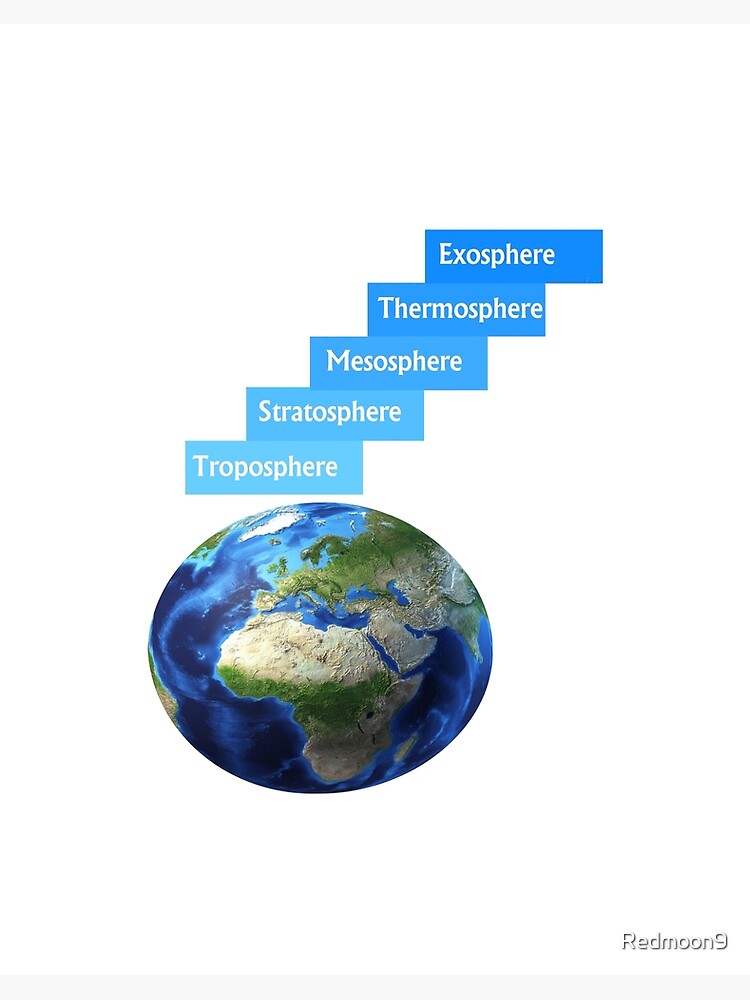This image is a detailed computer graphic illustrating the Earth's atmosphere, created by RedMoon9. At the bottom center of the picture is a two-dimensional rendering of the Earth, prominently featuring Africa in shades of green and brown, along with Europe and the Middle East. The surrounding oceans are depicted in dark and light blues. Above the globe are five sequentially arranged blocks, each labeled with a different atmospheric layer in ascending order. The lowest block, labeled "Troposphere," is in the lightest blue. Just diagonally above it to the right, a slightly darker blue block reads "Stratosphere." This pattern continues with "Mesosphere" in a moderately dark blue, "Thermosphere" in a darker blue, and "Exosphere" at the top in the darkest blue. Each block contains white lettering. Additionally, at the very bottom right of the image, the text "RedMoon9" appears, indicating the creator's branding.